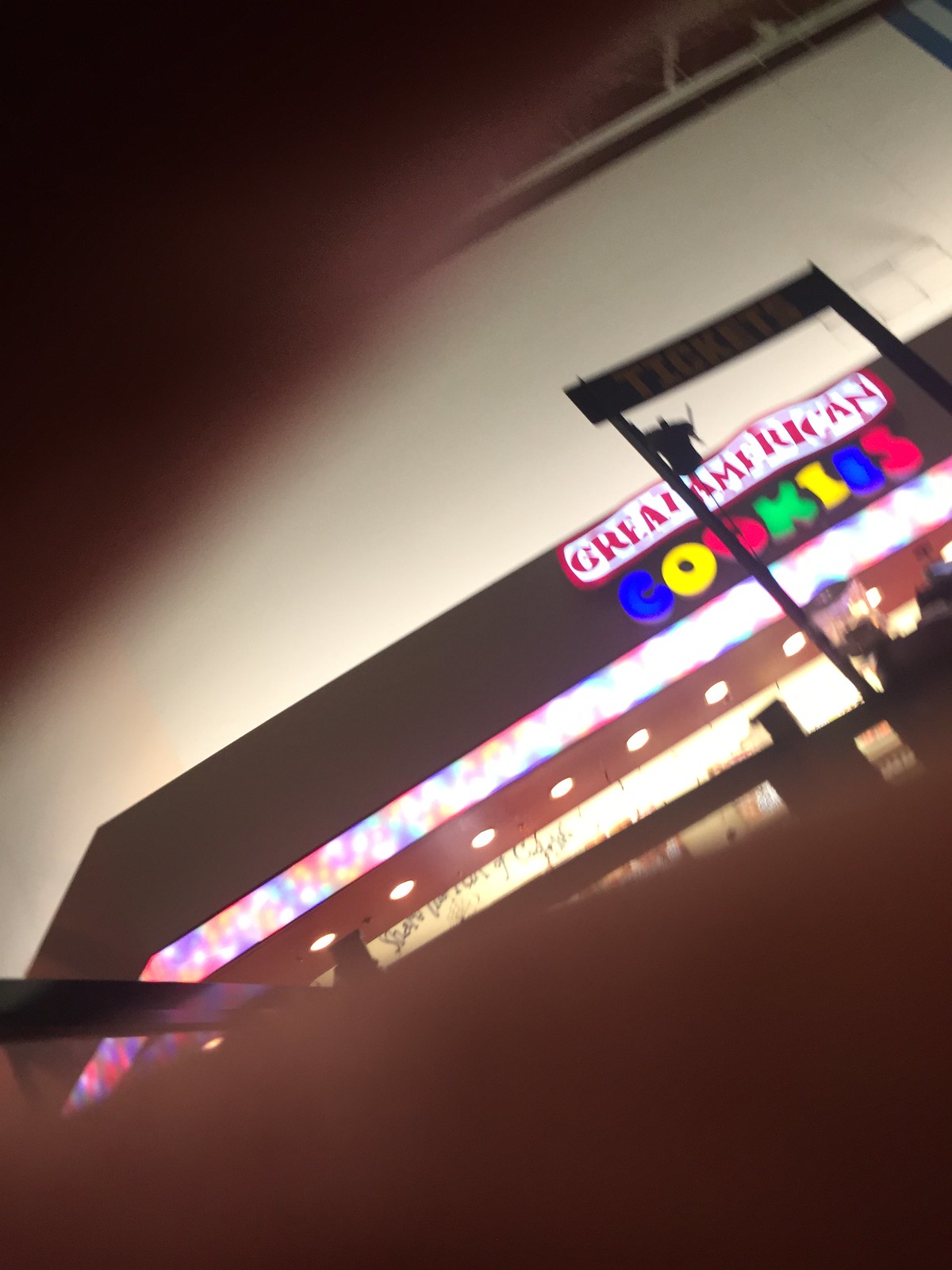The photograph appears to be taken in a mall and showcases the storefront of "Great American Cookies." The image is not well-focused, with noticeable blurriness due to the photographer's fingers partially covering the top left and bottom right corners of the lens, suggesting an accidental capture. In the clear portions of the picture, you can see a brightly illuminated neon sign that reads "Great American" in red on a white background, positioned above another sign that spells "Cookies" or "Cookios" with each letter in different colors: C in blue, O in yellow, second O in red, K in green, I in yellow, E or O in blue, and S in red. Additionally, extending above the cookie sign, there appears to be a ticket booth structure. Overall, the image gives an impression of an in-motion shot capturing part of the store's entryway.